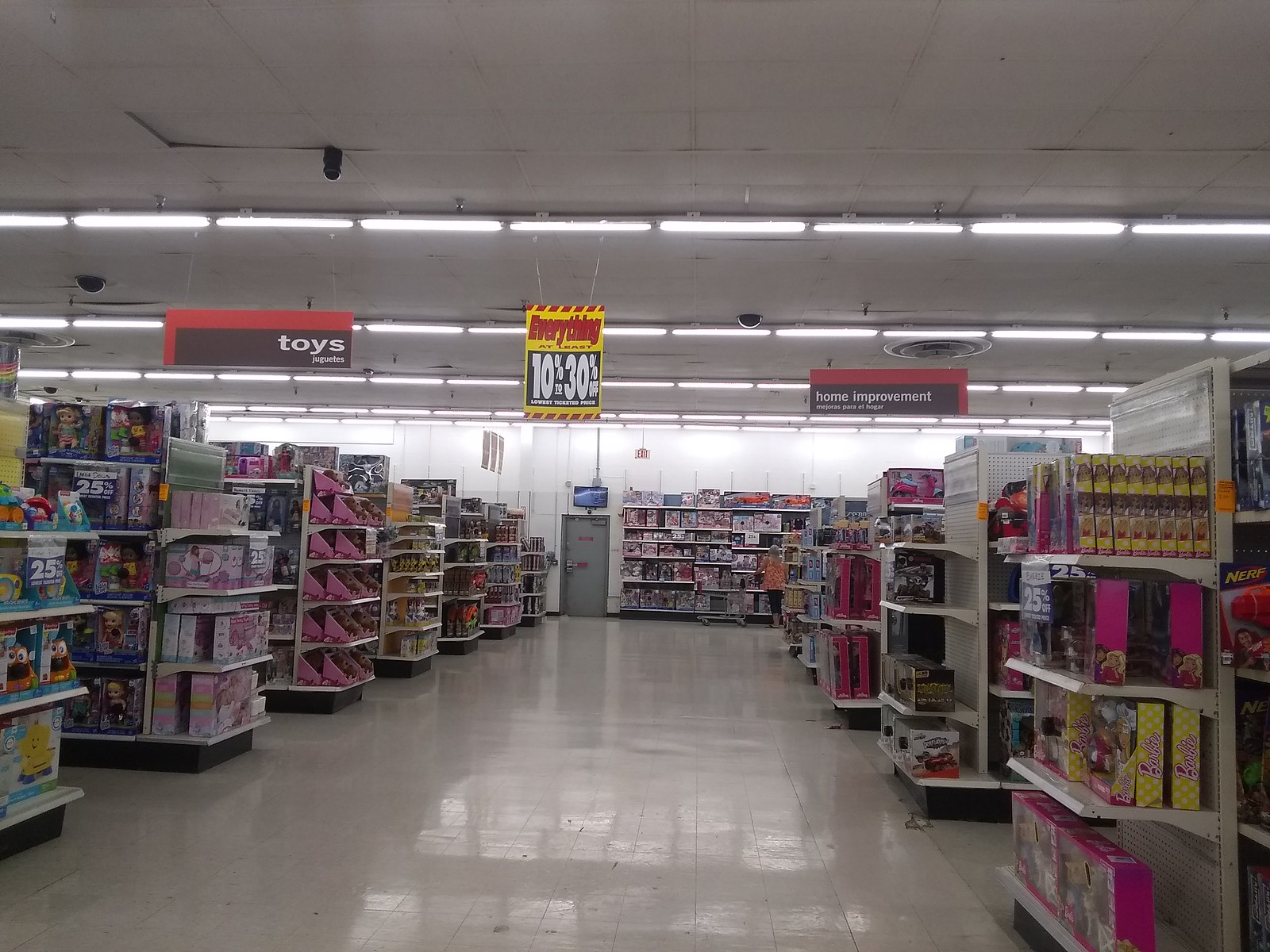The image captures a section of a retail store’s interior, focusing primarily on the ceiling area. Prominently visible are four black surveillance cameras mounted across the ceiling; three are relatively closer to the camera's viewpoint, while the fourth is positioned farther away in the back on the far left-hand side. Hanging from the ceiling are various signs, giving the image a lively yet organized appearance. One noticeable sign is brightly colored in yellow and red with bold white lettering, proclaiming, "Everything 10% to 30% off." Another directional sign, colored in a maroonish-reddish hue, indicates the section for "Toys." Opposite this, on the right side of the image, another sign points towards the "Home Improvement" section. The aisles below are densely stocked, and the shelves are filled with an assortment of boxed toys, making it evident that this part of the store is dedicated to children’s play items, amidst other household categories.